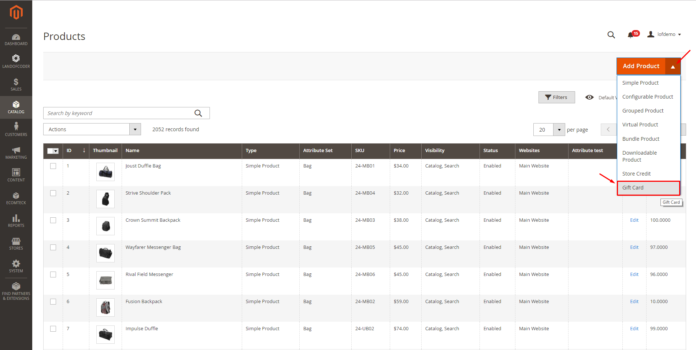This image appears to be a screenshot of a webpage displaying an inventory management or product listing interface. The page is blurry, making specific details difficult to read. Here is a detailed description of the visible elements:

The webpage has a black navigation ribbon along the left-hand side. The top of the white webpage has a header that reads "Products." On the right side of the top header, there are three icons: a search icon, a bell notification icon, and a user icon with a dropdown menu next to an unreadable username.

The central part of the page contains several sections. At the top, there is a light gray box with no visible text inside. Below this box, there is a "Search by keyword" option and an "Actions" dropdown menu. Beside this, the page indicates "2,052 records found."

A table occupies most of the page, divided into several columns and rows:

1. **First Column**: Contains a dropdown menu at the top and checkboxes down the length of seven rows. The purpose of these checkboxes is unclear due to the image's blurriness.
   
2. **ID Column**: Contains another dropdown menu at the top, with rows numbered from 1 to 7.

3. **Thumbnail Column**: Displays thumbnail images of various bags, such as backpacks, duffel bags, and messenger bags.

4. **Name Column**: Lists the names of the bags. Some identified names include:
   - Dow Duffel Bag
   - Strive Shoulder Pack
   - Crown Summit Backpack
   - Wayfarer Messenger Bag
   - Rival Field Messenger (uncertain)
   - Fusion Backpack
   - Impulse Duffel

5. **Type Column**: Describes all products as "Simple Products."

6. **Attribute Set Column**: Indicates all products belong to the "Bag" attribute set.

7. **SKU Column**: Each product has a SKU beginning with "24-M" followed by unreadable numbers except for some guesses:
   - 801 (first row)
   - 802 (seventh row)
   - Others vary but are unclear

8. **Price Column**: Displays prices for each product, with some examples being $34, $32, $38, $45, and $74.

9. **Visibility Column**: Indicates "Catalog Search" for all listed products.

10. **Status Column**: Shows that the status of each product is "Enabled."

11. **Websites Column**: Lists "Main Website" for all products.

12. **Attributes List Column**: Appears to be blank for all rows.

There are two more columns obscured by a pop-up menu on the right side of the page. The visible text in the pop-up reads "Add Product" with multiple options in a dropdown menu, such as "Simple Product," "Configurable Product," "Grouped Product," "Virtual Product," "Bundled Product," and "Gift Card" (the selected option).

Moreover, starting from the third row in the final visible columns, there are links labeled "Edit" next to monetary values like $100,000, $97,000, $96,000, and $10,000, though not all numbers are decipherable.